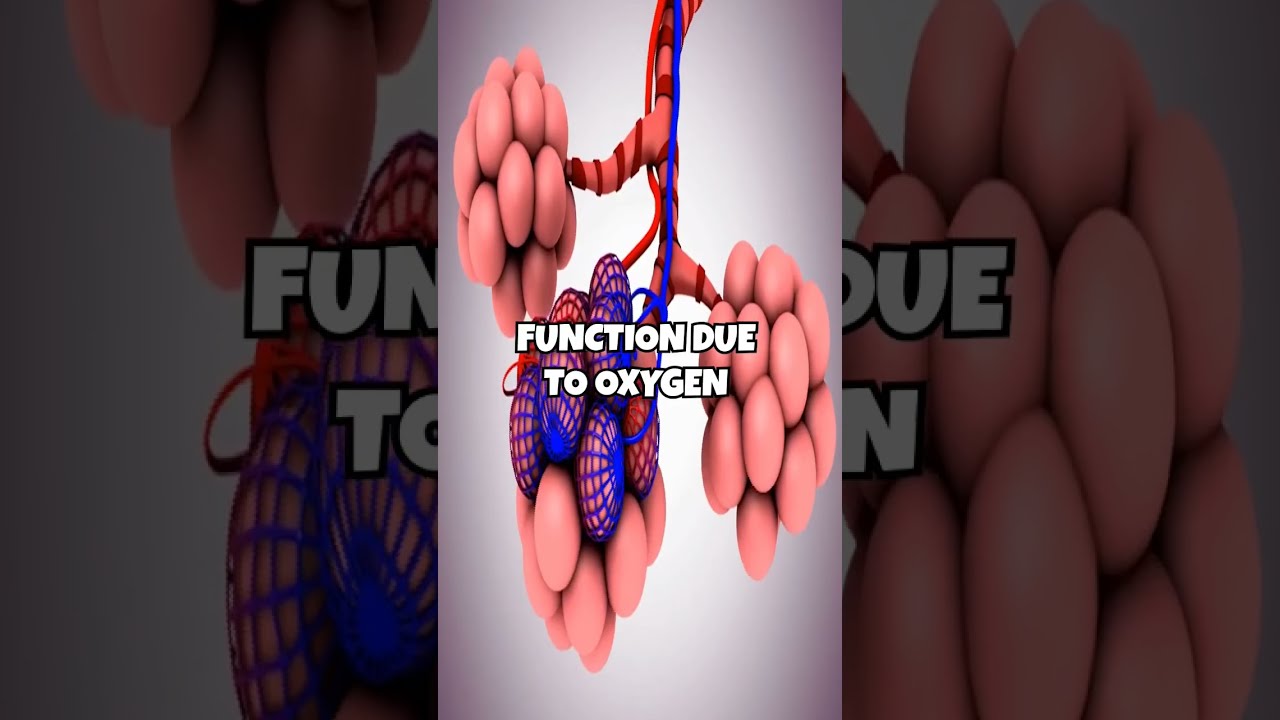This horizontal rectangular image is a detailed 3D computer-generated illustration depicting organic material, possibly cells. The background is predominantly a close-up of the central element, which is rendered as a vertical rectangle with a grayish gradient, more whitish at the center to highlight the details. Bold white text with black borders runs across the center, reading "function due to oxygen."

The middle section of the illustration is split into three panels. The central panel showcases a structure resembling a branching tree, with clusters of oval-shaped pink entities at the ends of its branches, suggesting some sort of cellular clusters or molecules. Above and below the text, these clusters appear again, with the one below being partially enclosed in a blue net-like structure. 

The left panel provides a close-up of the blue-netted cluster against a darker charcoal gray background, while the right panel offers a close-up of the pink cluster against a similarly darkened background. The charcoal backgrounds in the left and right panels contrast sharply with the central imagery, accentuating the detailed organic forms against a more subdued backdrop.